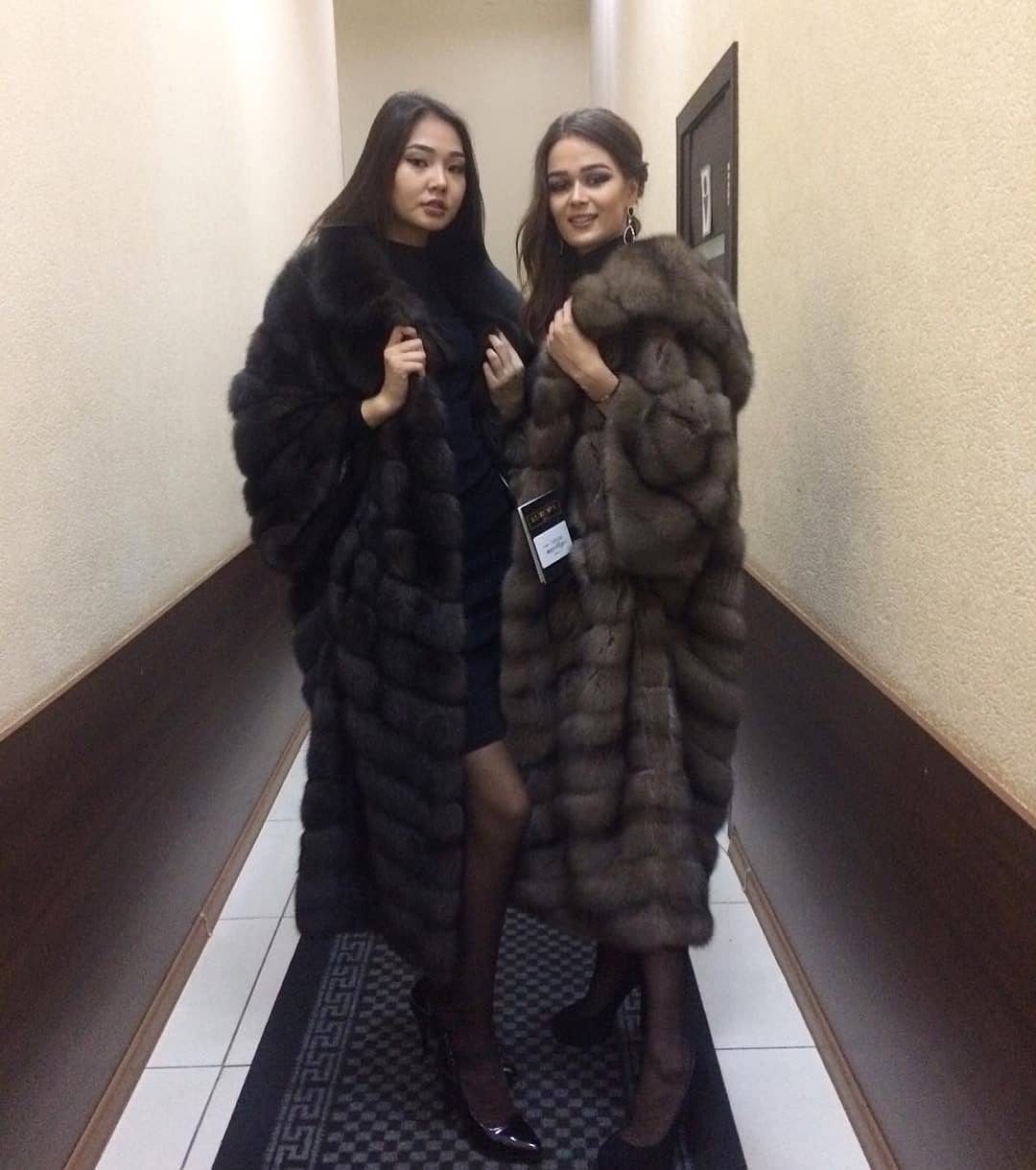The image features two young women standing in a narrow hallway, posing mid-smile for the photo. Both women have medium skin tones and long black hair flowing behind them. They are dressed in luxurious dark fur coats that reach to about six inches above their ankles, paired with black heels and black hose. The woman on the left has both hands holding the front of her coat, drawing attention to its plush texture. The woman on the right is slightly turned, with one hand holding her coat in a similar fashion, and the other hand possibly interacting with a paper or tag attached to her fur coat. 

The hallway is characterized by cream-colored walls with brown paneling at the bottom and white tile flooring, accentuated by a maroon floor runner. Additionally, there is beige-y pink wall color and a door situated behind the women on the right side of the hallway. The scene captures a moment of poised elegance and subtle sophistication.